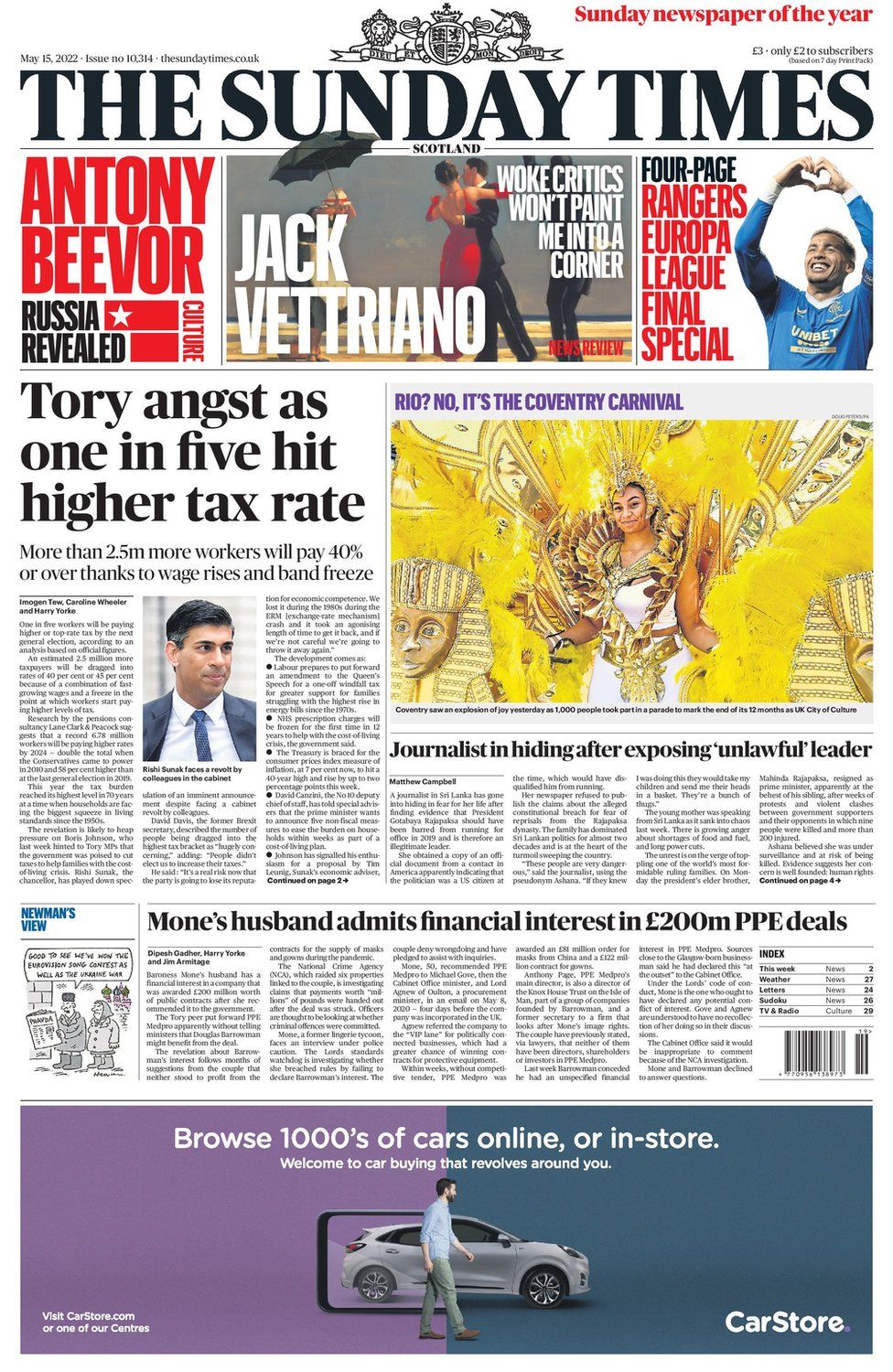This is a detailed caption to provide an accurate and engaging description of the image you described:

"A screenshot of the front page of the Sunday Times, presumably taken from its online edition, is showcased. Dominating the top of the page, the newspaper's name, 'The Sunday Times,' is boldly displayed in large black letters stretching from the left to the right. Above the word 'Sunday,' a subtle and intricate gray illustration, resembling a coat of arms, adds a touch of elegance. Just below the masthead, a striking photograph captures a moment of ballroom dancing. The image features a man in a black suit and a woman in a flowing red sleeveless gown, dancing gracefully. Accompanying the photograph, text in white font reads 'Jack Vettriano' on the left and 'Woke Critics Won't Paint Me Into a Corner' on the right. To the left of the main photograph, there is a visually captivating drawing set against a yellow background, depicting a performing artist adorned in an ornate gown, vest, jacket, and a golden headpiece. Flanking this central figure are stylized golden figures reminiscent of King Tut and Egyptian art. The newspaper also features a headline on the far left in black font that reads 'Tory Angst Has One in Five Hit Higher Tax Rate.' Below this headline is the beginning of a lengthy article, although the font is too small to decipher the text from the screenshot."